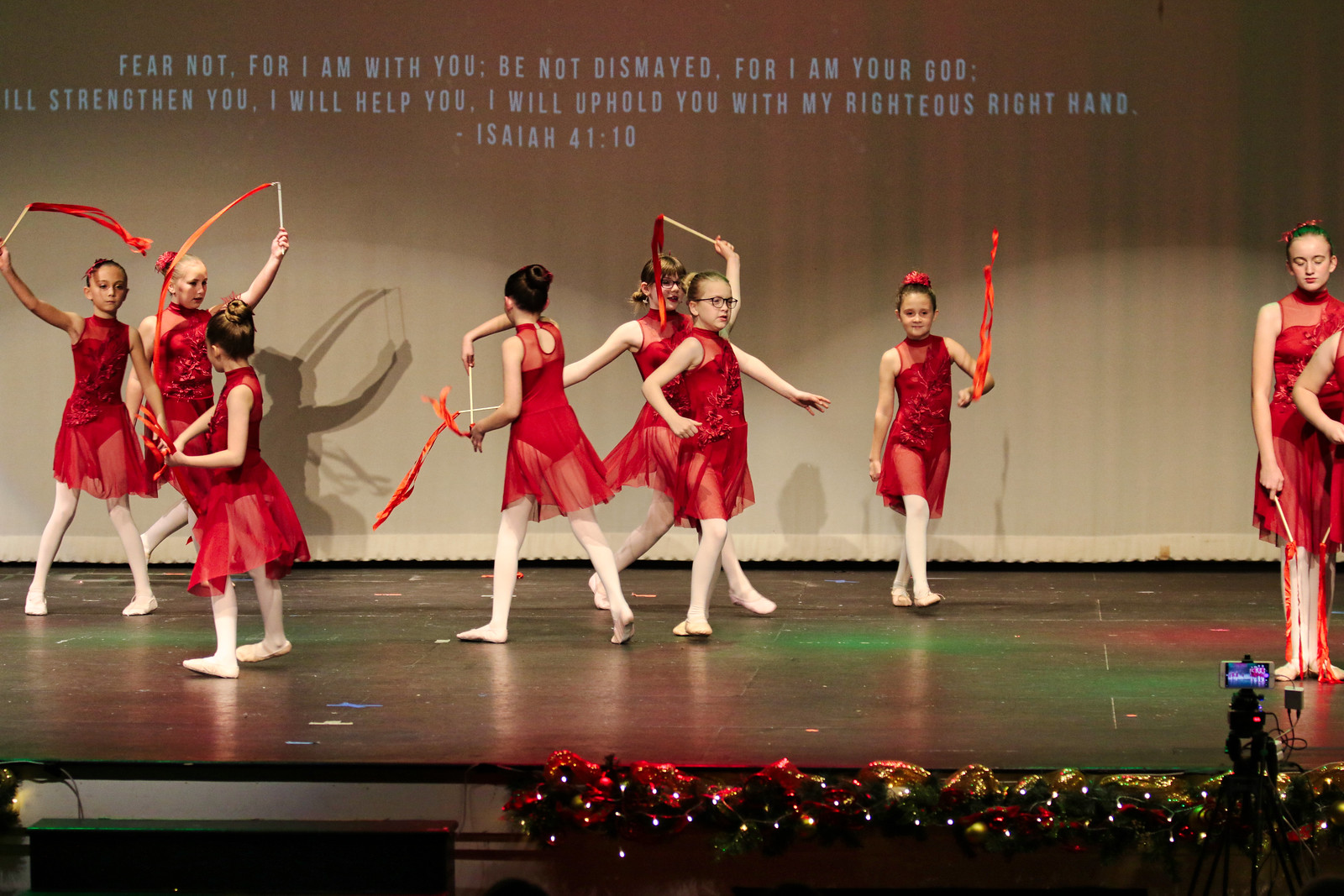In this vibrant stage performance, a group of nine young girls, possibly around 10 to 11 years old, are exuberantly waving red ribbons attached to white sticks, creating a synchronized display reminiscent of ballet or gymnastics. Each girl is dressed in a sleeveless red dress paired with white tights and ballerina shoes, with their hair neatly pulled up. The stage itself features a striking blacktop arch, adorned at the front with a festive garland intertwined with white LED lights and gold ribbons, suggesting a Christmas theme. Behind the girls, a pristine white curtain serves as the backdrop, displaying in bold white capital text, the comforting biblical verse from Isaiah 41:10: "Fear not, for I am with you; be not dismayed, for I am your God. I will strengthen you, I will help you, I will uphold you with my righteous right hand." The stage's front is white, and lights in red and green hues are reflected across it, further amplifying the holiday atmosphere. To the bottom right, a camera on a stand captures this enchanting moment, preserving the joyous spirit of the event.